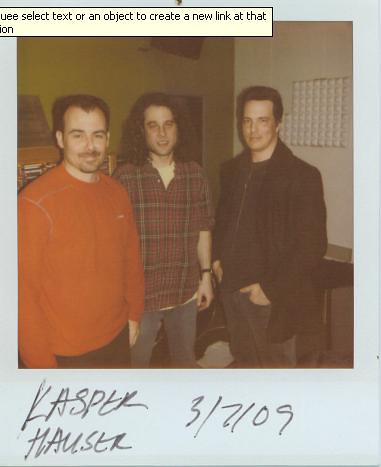A slightly fuzzy, faded Polaroid with a distinct white border features three men standing in a room with white walls and various objects, possibly tables, wall hangings, and a bookshelf, in the background. The Polaroid has handwritten text at the bottom that reads "Casper Hauser, 3709." The man on the left, a white individual with short dark hair, a faint mustache, and a goatee, is wearing an orange sweatshirt and dark pants. He is smiling at the camera. The center man, also white and clean-shaven, has long, shoulder-length hair. He is dressed in a red and black plaid shirt over a white t-shirt, wearing jeans and a wristwatch, and is smiling as well. The man on the right, another white individual with short to medium-length slicked-back hair and neatly combed black hair, wears a black overcoat over a black zip-up shirt, dark pants, and has his hands in his pockets. In the upper left corner of the image, there is an overlaid box containing partially visible text that includes "select text or an object to create a new link at that." The overall atmosphere suggests an informal gathering captured in a snapshot from the past.